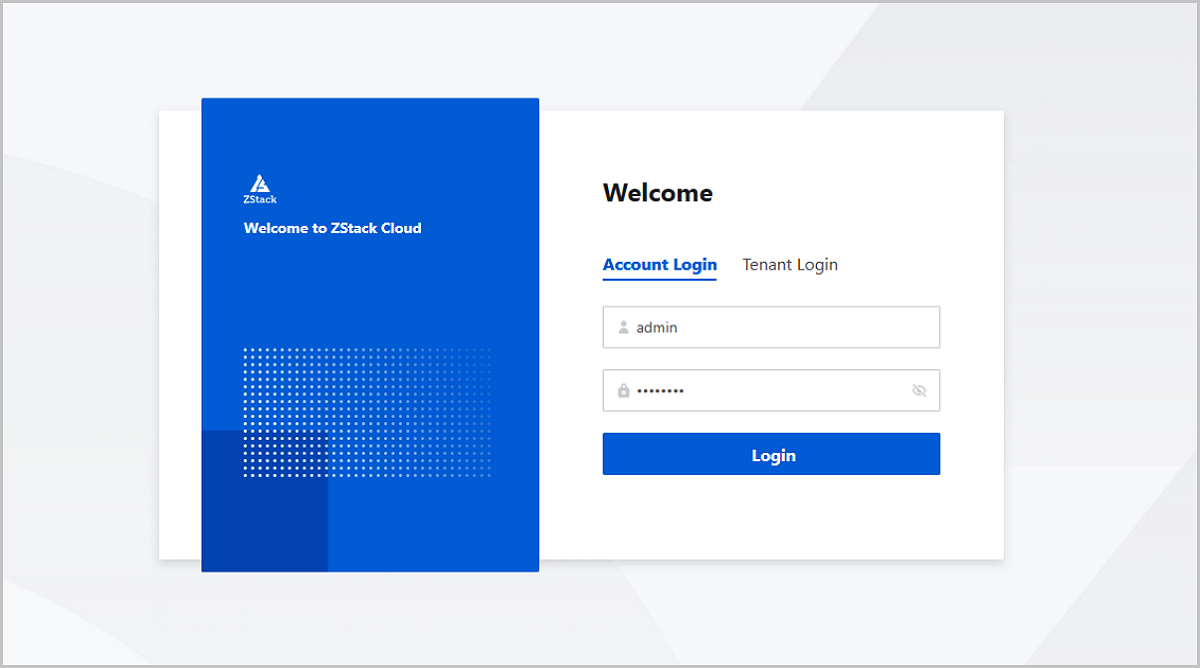The image features a login interface for "Z Stack Cloud." 

The background of the image is a light blue color, framed with a darker gray outline. Within the frame is a white central box. On the left side of this white box is a blue square containing a white triangle with the text "Z Stack" written inside the triangle in white lettering. Below this, it says "Welcome to Z Stack Cloud," followed by a series of small white dots. In the bottom left corner of the blue square, there is a smaller, darker blue box.

On the right side of the white central box, the background remains white. At the top, bold black text reads "Welcome." Below this, blue text that says "Account Login" is underlined in blue. To the right of "Account Login," it says "Tenant Login."

Further down, there is a gray box featuring an icon of a person and the word "admin" in gray letters beneath it. Next to this, there is a lock icon accompanied by a series of dots. At the bottom of this section, there is a blue login button with white text that says "Login."

The color scheme throughout the image includes only blue, white, gray, and black. This carefully designed layout serves as the login interface for "Welcome to Z Stack Cloud."